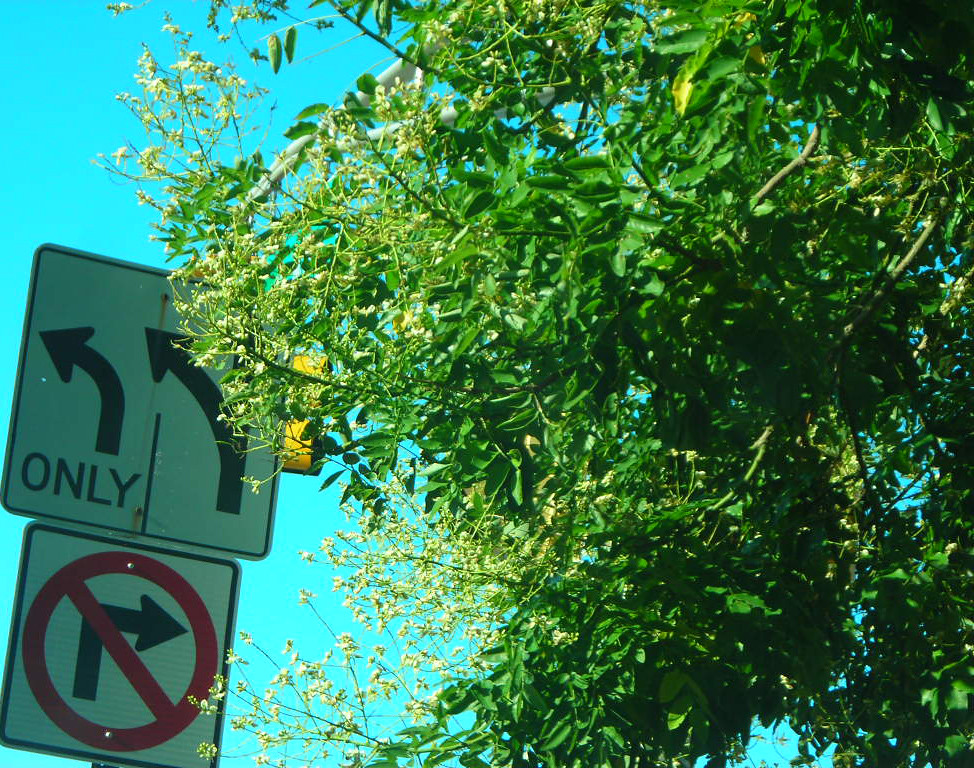The image features a lush arrangement of green leaves, predominantly on the right side, with varying shades of green—from darker hues on the right to lighter greens on the left. Small branches intertwine through the foliage, some even displaying delicate yellow flowers. On the left-hand side, there is a sign with an arrow indicating a left turn. Adjacent to it, another sign on the right shows an arrow pointing both left and forward. Below these, a white sign with a big red slash mark indicates a prohibition, likely concerning a right turn. In the background, a yellow traffic light is faintly visible through the dense clusters of leaves, adding a touch of urban context to the verdant scene.